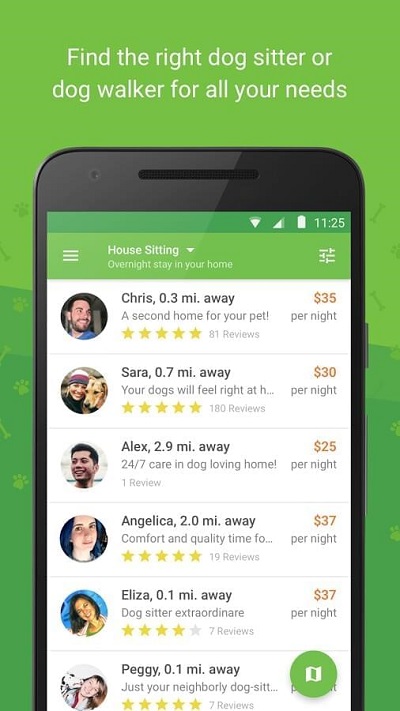The image features a black cell phone set against a vibrant green background. At the top of the image, white text reads, "Find the right dog sitter or dog walker for all your needs." Below this text, the cell phone display is visible, showing a pet care application.

On the screen, the app's interface has a green header with white text stating, "House sitting, overnight stay in your home." Below the header, search results for pet sitters are displayed, listing six profiles in total.

The first profile features a circular, thumbnail photograph of a white man with dark hair, a beard, and a mustache. The profile information reads: "Chris, 0.3 miles away. A second home for your pet. Five stars, 81 reviews, $35 per night."

The second profile shows a white woman wearing a knit hat, next to a tan-colored dog. The profile reads: "Sarah, 0.7 miles away. Your dogs will feel right at H... Five stars, 180 reviews, $30 per night."

Four additional profiles follow in a similar format, each with a circular photo and detailed information about the pet sitter.

In the bottom right corner of the screen, there is a green circular button with an indiscernible square-shaped symbol, possibly indicating a chat or contact feature.